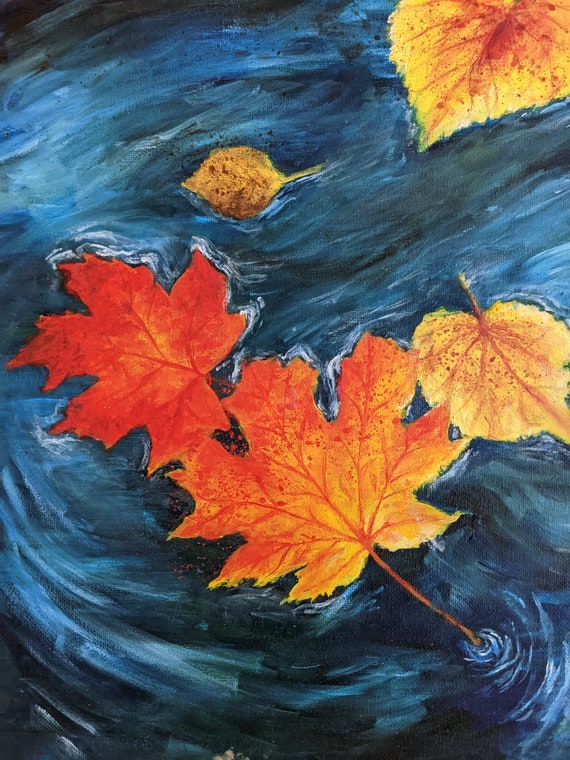This vibrant oil-based painting features a dynamic scene of autumn leaves floating on swirling water. The predominant colors in the painting are rich blues and blacks, accented with bright oranges and yellows to highlight the fall foliage. The water, illustrated with deep, swirling blue patterns and touches of black, gives a sense of depth, with white outlines around the leaves enhancing the perception of motion. The image showcases various types of leaves—most notably two maple leaves with five and six points, colored in vivid yellow-orange hues, centrally positioned. Alongside them, three other leaves with elliptical, teardrop shapes, displaying a mix of reddish and yellow tones with brown spots and prominent veins, add diversity to the composition. A small brown leaf hovers above the top maple leaf, contributing to the complexity of the scene. The overall depiction captures the essence of autumn, with the leaves seemingly having drifted from nearby trees, now floating and swirling on the dynamic, dark blue water below.